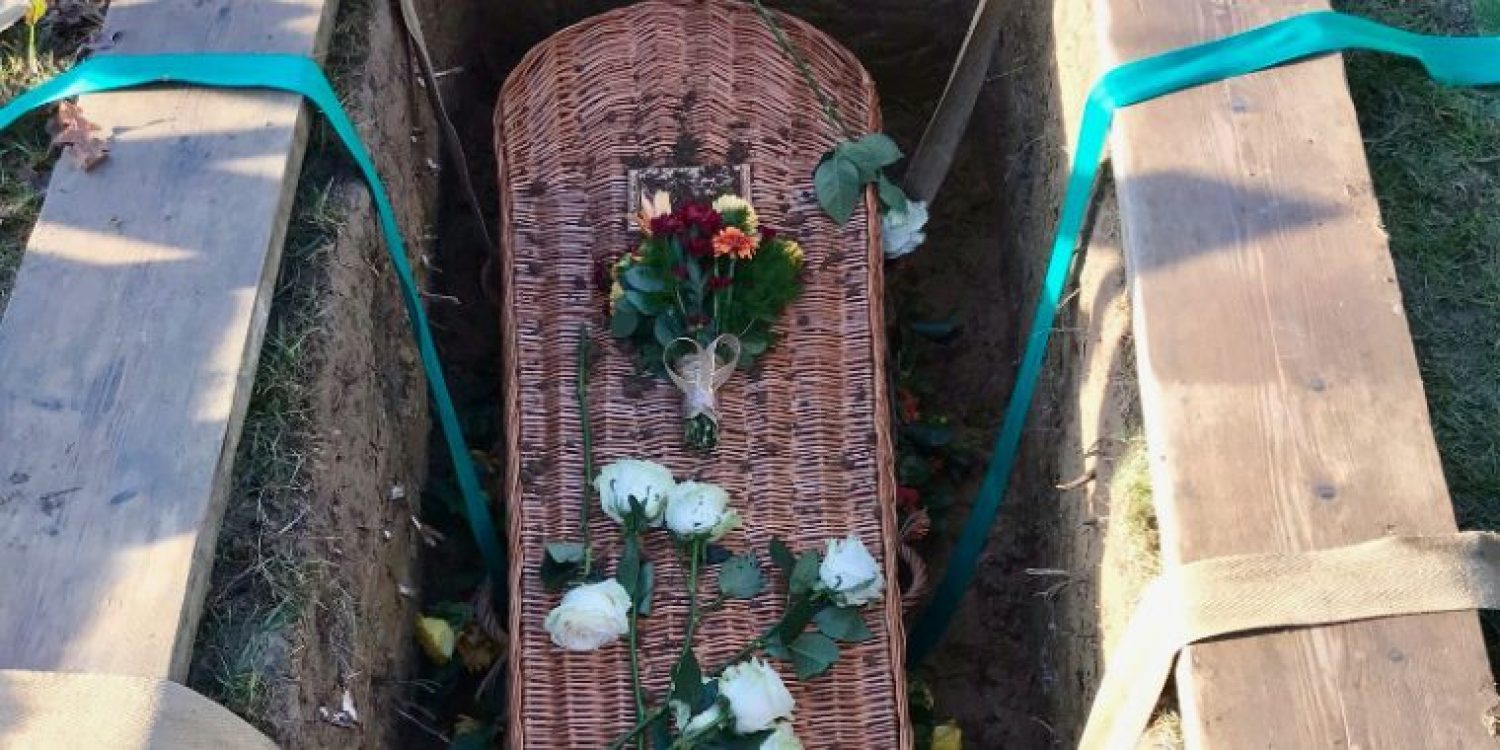The image depicts a solemn scene of a wicker coffin being carefully lowered into a grave. Surrounding the grave, grass is visible along the far edges, while two wooden planks rest on either side of the hole, supporting the green straps that guide the descent of the coffin. The wicker coffin, appearing almost at the bottom of the grave, is adorned with a bouquet of dark burgundy, orange, and yellow flowers tied with a light-colored ribbon at its center. Scattered atop the coffin are seven white roses, alongside bits of dirt. Additional flowers, including some yellow roses, have fallen to the sides. These small floral tributes contrast with the earthy tones of the grave, adding a poignant touch to the scene.